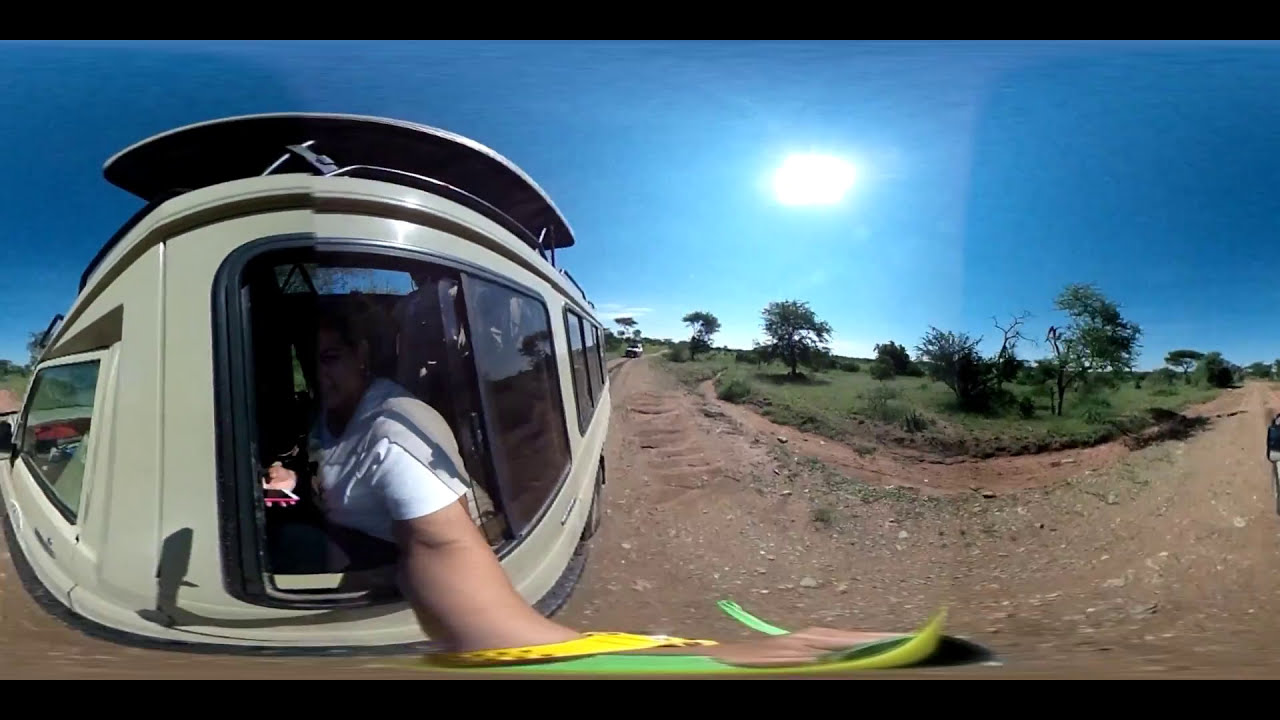In this panoramic image, a person, possibly a woman, is seen driving an olive-colored van down a long dirt road. Her left hand is extended outside the vehicle, potentially taking a selfie or using the camera to capture this expansive scene. The van appears large and has a sliding window that has been opened to the right side. The individual is wearing a white short-sleeve t-shirt, and there are yellow and lime green papers or items visible near her arm inside the vehicle. The atmosphere appears quite warm, emphasized by the intense blue sky and the bright sun situated almost in the center-right of the photograph, indicating a hot day. The landscape to the right is marked by lush greenery and trees. Another vehicle can be seen in the background, seemingly traveling in the opposite direction. This vivid image, with its high-definition resolution and wide-angle distortion that may resemble a fisheye lens effect, captures the essence of a sunlit adventure on an unpaved, dusty path.